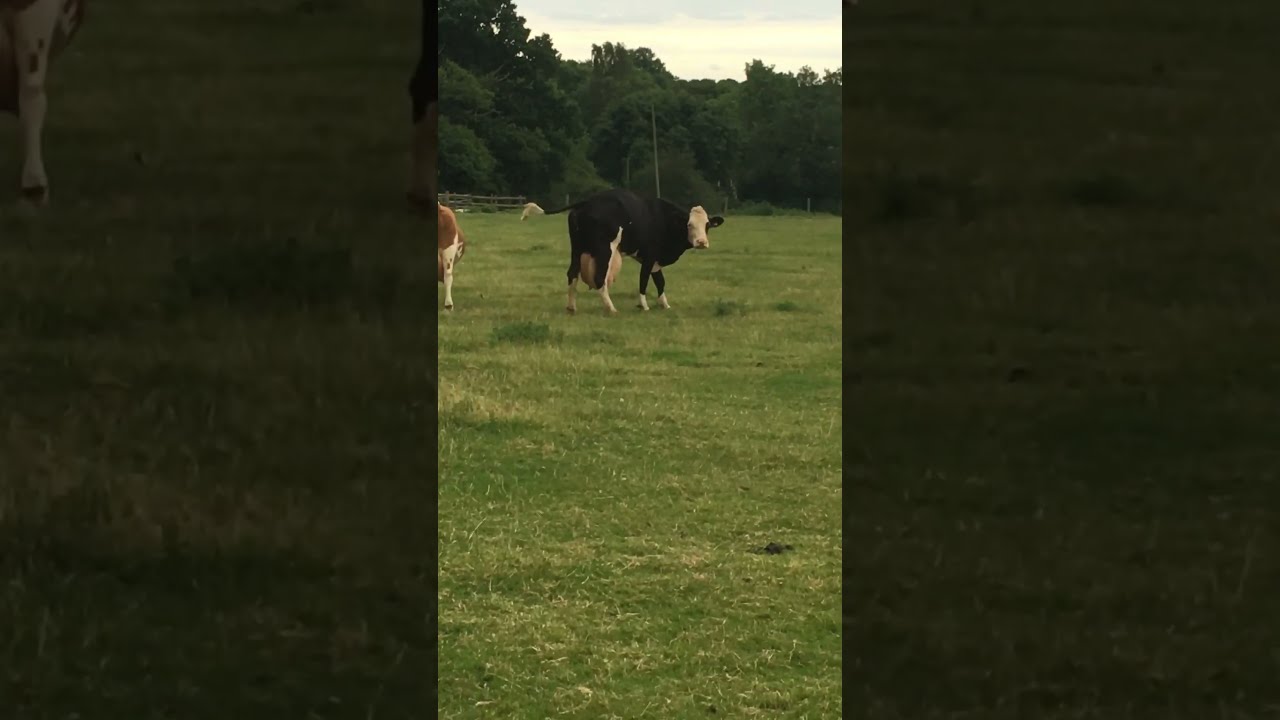A detailed image showcases two cows standing in a grassy field under a dull, grayish sky. The central focus is a black cow with a distinctive white head and exceptionally full, nearly spherical udders, illustrating its readiness for milking. Surrounding this cow, the patchy grass ranges from a vibrant green to light brown, adding texture to the scene. In the background, a dense line of rich, dark green trees serves as a contrasting backdrop. To the left of the image, the partial view of a brown and white cow is noticeable, though only its white legs and a bit of its rump are visible, suggesting it is slightly outside the frame's main focus. This composition is artfully captured within a photograph that occupies the center of a larger frame. The surrounding sections of the larger frame feature zoomed-in segments of the primary image, overlaid with a dark, opaque tint. The right side displays a close-up of the green and brown grass, while the left side showcases a detailed view of the brown cow's white leg. The overall presentation gives a cohesive yet detailed perspective of a tranquil pastoral setting.